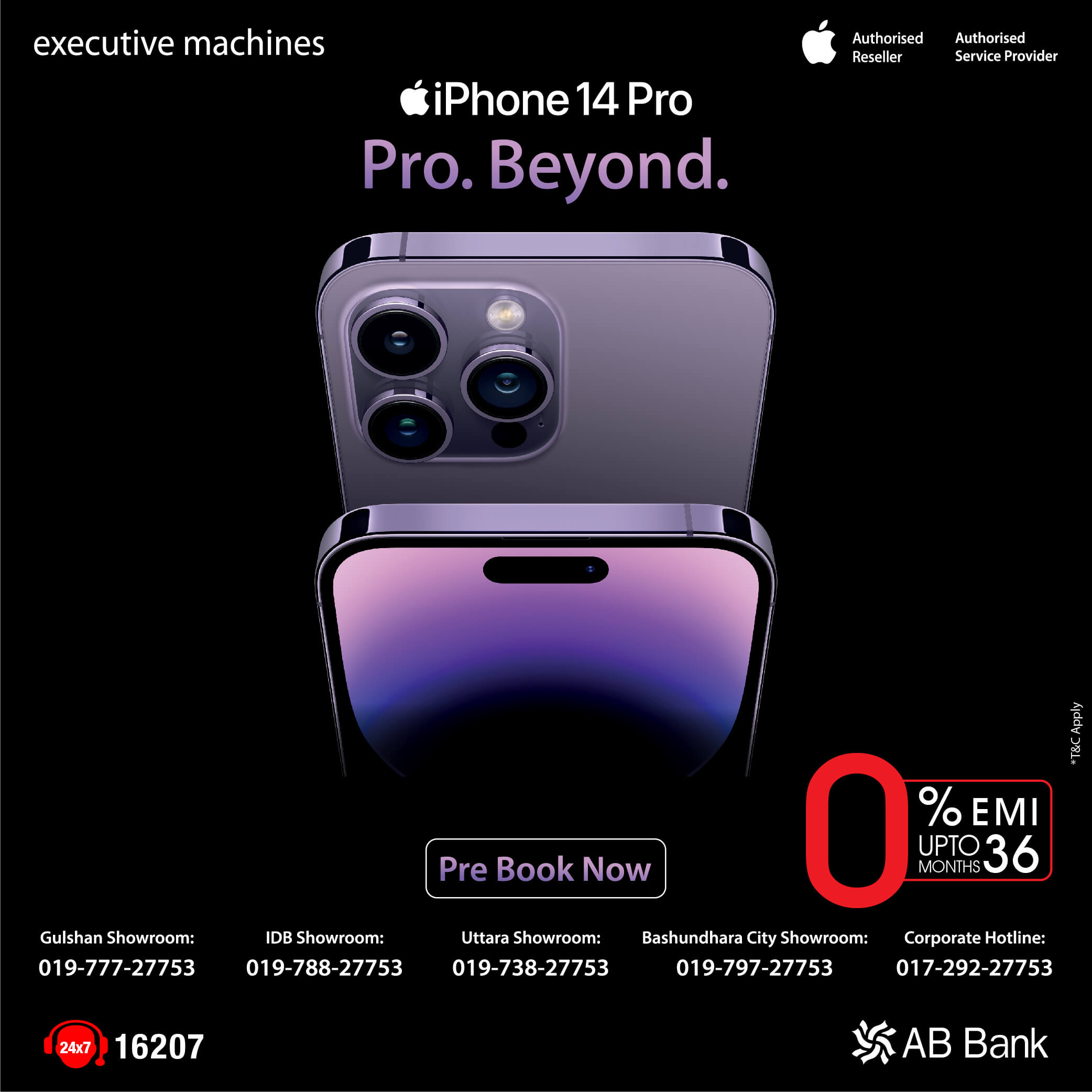Top left is the logo for Executive Machines, while the top right displays logos for Apple Authorized Reseller and Apple Authorized Service Provider. In the center, there’s a vibrant image of a purple Apple iPhone 14 Pro showcasing its three rear cameras arranged in a triangular configuration, along with a flash and some elegant trim. The iPhone stands out with a gradient color transition from purple to blue and finally to black towards the bottom.

Below the phone, there's a call to action stating, "Pre-book Now," accompanied by an offer that reads "0% EMI up to 36 months" in red text. 

Alongside, various contact numbers for showrooms are listed:

- Monolith showroom: 019-777-27753
- Goldstrand showroom: 019-78-27753 
- Altara showroom: 019-73-27753 
- Corporate hotline: 017-219-27753 

Additionally, the bottom left corner features a "24/7 hotline: 16207", and the bottom right corner exhibits wavy symbols with an AB Bank logo. The entire design is set against a sleek black background, amplifying the prominence of the vibrant elements.